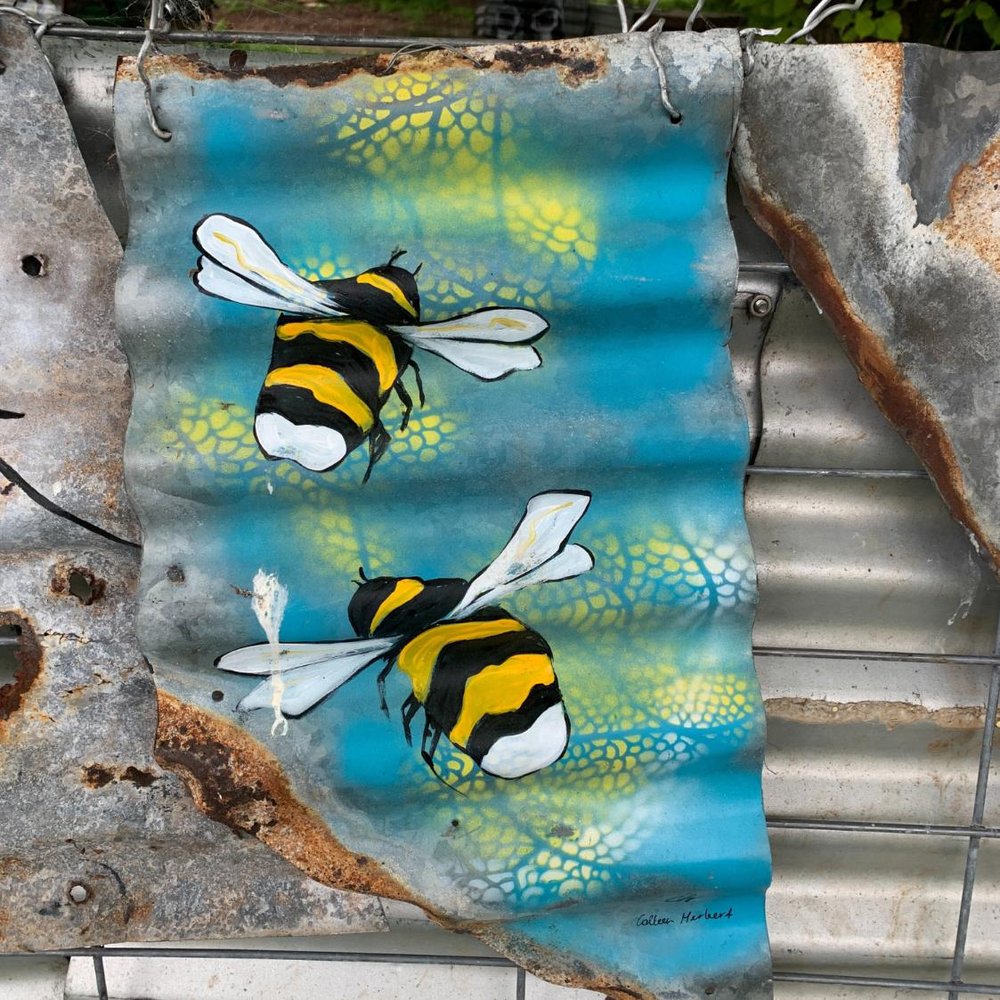This detailed image captures a piece of graffiti art adorning a metallic sheet, which is hung against a silver, rust-patched shutter using thin horizontal wires. The metallic sheet, itself also showing signs of rust, has been creatively transformed with vivid spray paint. The background of the artwork features a striking blue sky interspersed with a yellow, scaly honeycomb pattern that traverses from the top center down towards the bottom right corner. Centrally positioned, two large bumblebees, with classic black and yellow stripes and four delicate white wings each, are depicted in flight. The artist's signature, "Colleen Herbert," is neatly inscribed in the lower right corner, testament to the skill and imaginative vision behind this outdoor installation.